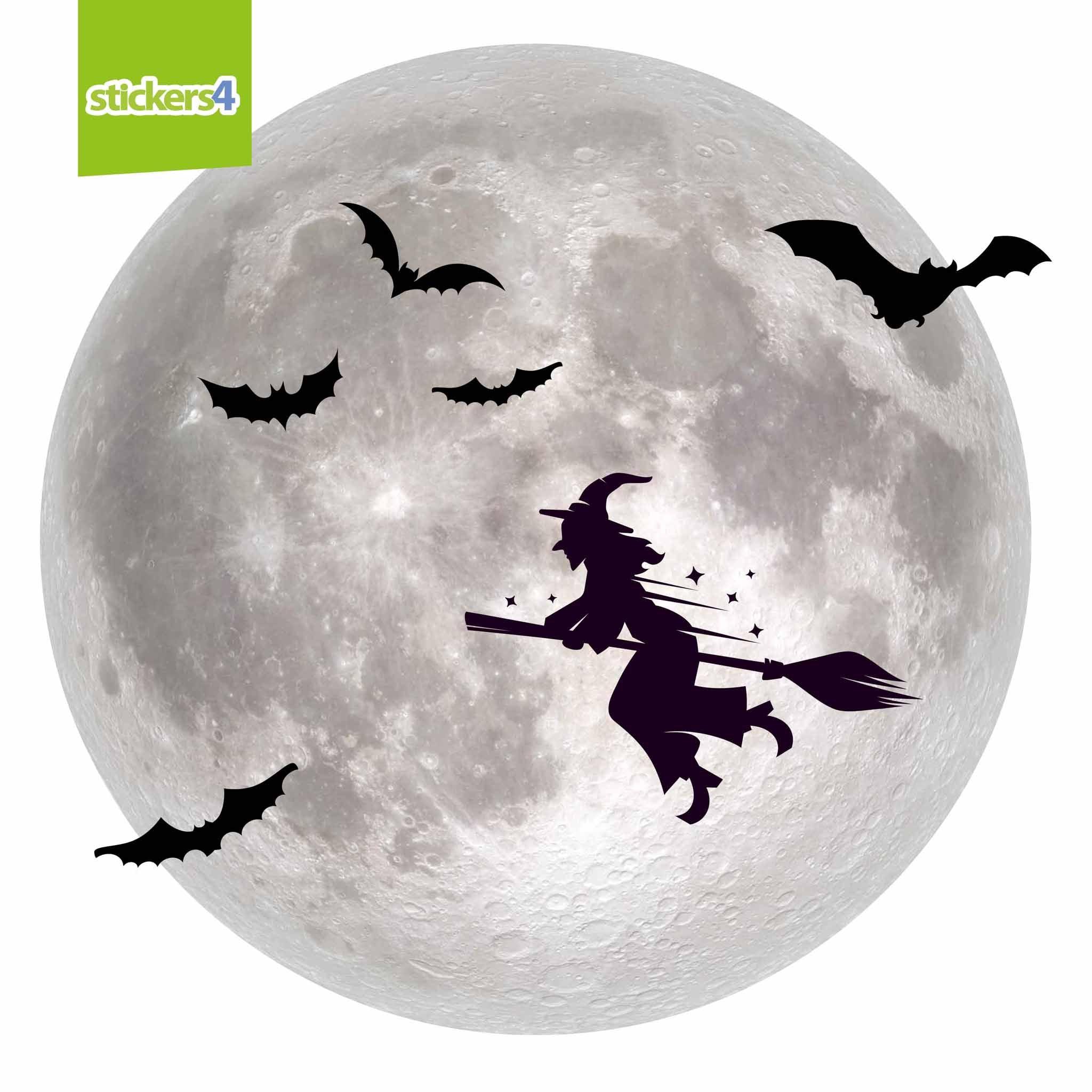The image features a realistically textured moon with a grayish surface and white ridges and bumps, set against a white background. In the top left corner, there's a neon green square, sliced at an angle, containing the word "stickers" in green font and the number "4" in blue. Arranged in front of the moon is a sticker pack, including a black silhouette of a witch riding a broom from right to left. The witch is detailed with a pointed hat, long nose, loose pants or robe, and boots, with six star-like structures trailing around her suggesting magical twinkling. Additionally, there are five bats in flight, varying in size and distance, positioned below and around the witch, contributing to the spooky Halloween theme.